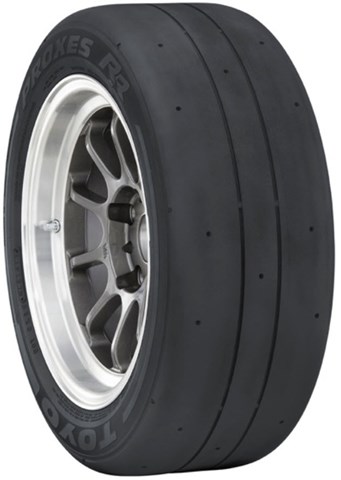The image depicts a single, black Toyo tire mounted on a brushed aluminum, multi-spoke rim. The view is isometric, so you cannot get a straight-on perspective of the tire's size, but you can identify details from the sidewall text, which reads "Proxes RR" at the top and "Toyo" at the bottom. The tire is stationary and angled such that the rim, which has an estimated 10-15 spokes, faces slightly to the left. The tire itself features two indented lines running down its smooth surface along with several small, crater-like holes. The side of the tire exhibits some grey, indented lettering, and the tire's sections include two thicker black portions flanking a thinner central section with a straight tread in the middle. There are also two black knobs visible near the center of the rim.